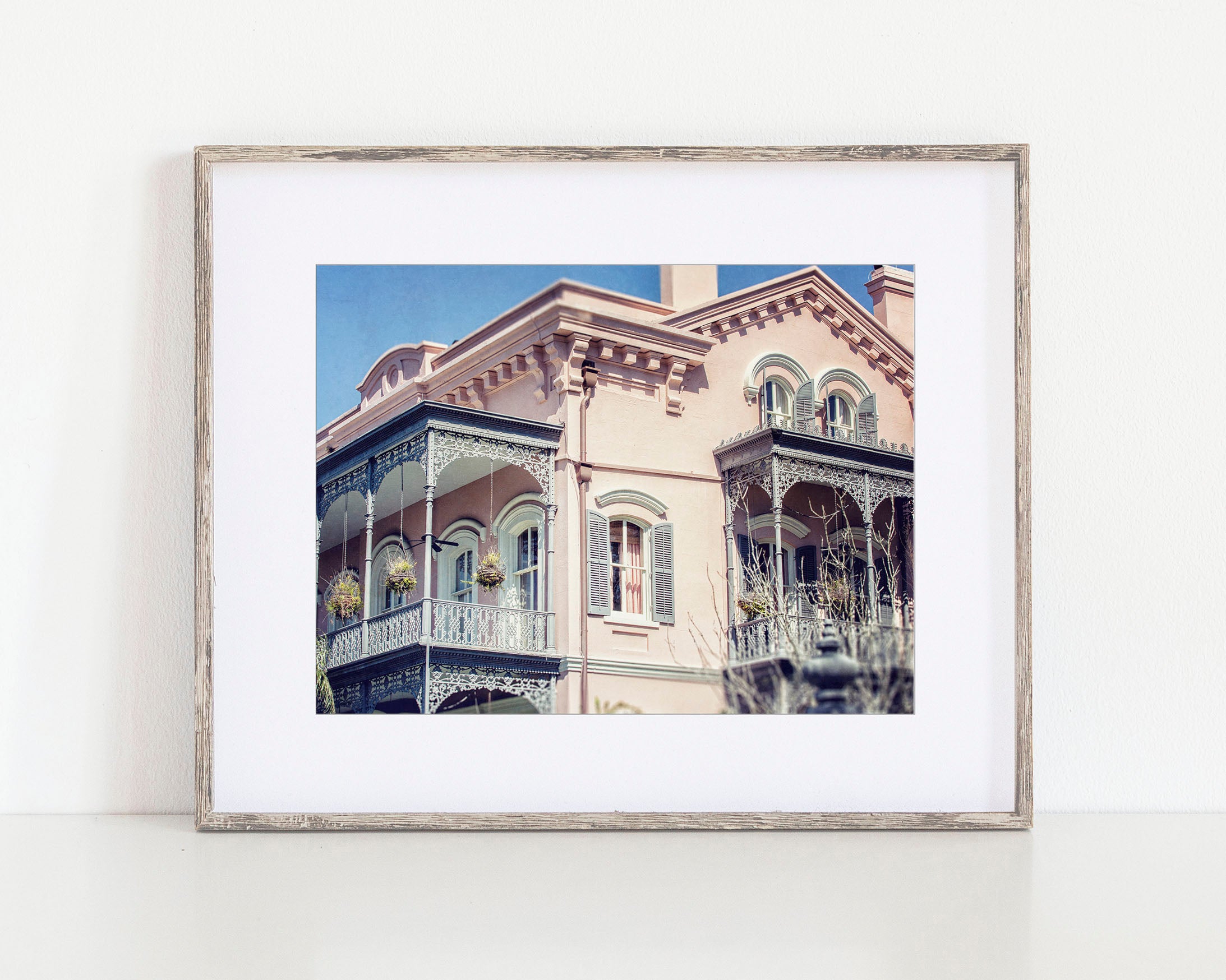The image depicts a photograph of a pink, three-story building, evocative of Southern architecture typically seen in New Orleans or Charleston, South Carolina. The building, which might function as a large residence or hotel, features an old design that's likely a couple of hundred years old. It boasts elaborate wooden balconies and ornate columns at the roofline, with intricate carved designs adorning the awnings. The balconies on the second floor are decorated with hanging plants, and additional balconies mirror this ornate style. Arched windows with green shutters are prominent, complemented by a detailed white banister around the second-floor veranda, which contains three windows. There are a few trees with leaves visible in the lower right quadrant against a blue sky backdrop. The photograph is framed with a wooden frame and a white mat, set against a white background, suggesting it might be displayed in a museum or gallery.